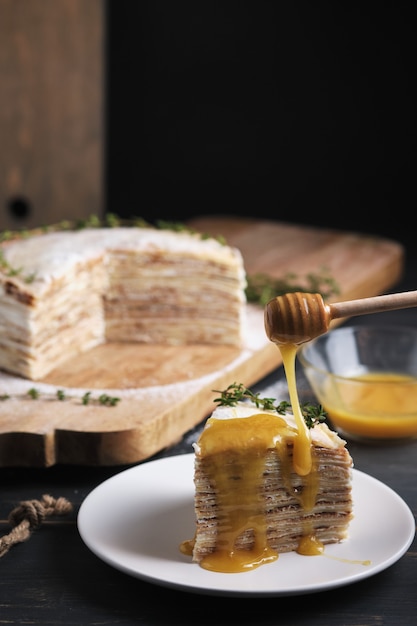In this photograph, we see a detailed close-up of a multi-layered cake slice resting on a white plate, which is placed on a dark grayish-blue table. The cake slice features alternating light brown and dark brown layers, topped with a white layer that could be icing or powdered sugar. A gold, caramel-like sauce is being drizzled over the cake from a honey dipper, suggesting a sweet enhancement to the dessert.

To the right of the cake slice sits a bowl containing the same drizzling mixture, hinting at honey mixed with another substance due to its cloudy yellow hue. A sprig of thyme is delicately placed on top of the cake, adding a touch of greenery to the presentation.

In the background, we can see the rest of the cake on a light brown wooden cutting board, indicating that a slice has been taken out. This composition is set against a backdrop that transitions from dark brown on the left to black on the right, emphasizing the cake and its intricate details.